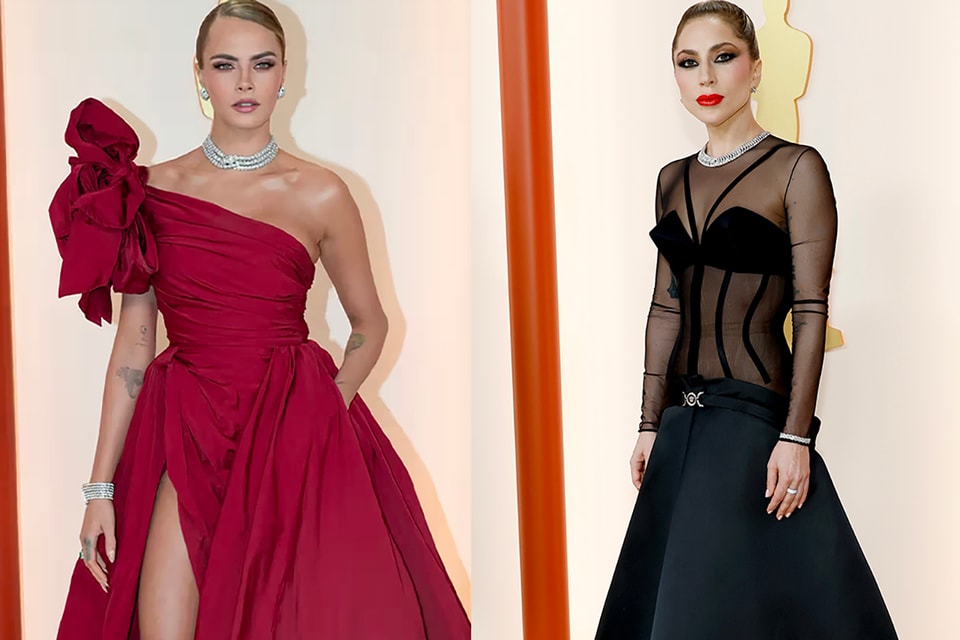The image features two prominent women attending what appears to be a red carpet event, possibly the Oscars, as suggested by the visible golden Oscar trophy in the background. On the left, Cara Delevingne dazzles in a strapless, crimson red dress with an elaborate bow on her right shoulder. Her dress has a dramatic slit revealing her right leg, and she accessorizes with an array of jewelry including a large diamond bracelet, diamond earrings, and a multi-layered pearl necklace. Her light brown hair is neatly pulled back and parted to the side, revealing tattoos on both her forearms.

On the right, Lady Gaga makes a striking appearance in a black, sheer long-sleeve dress. The sheer fabric extends from the sleeves to the upper part of the dress, with opaque black cups covering her breasts, along with two black stripes that run over her shoulders. A black skirt completes her elegant yet edgy look, accentuated by a belt adorned with a diamond centerpiece. Gaga complements her ensemble with bright red lipstick, dark eye makeup, and an elegant necklace. The attention to detail in both outfits and accessories underscores the sophistication and glamour of the event.